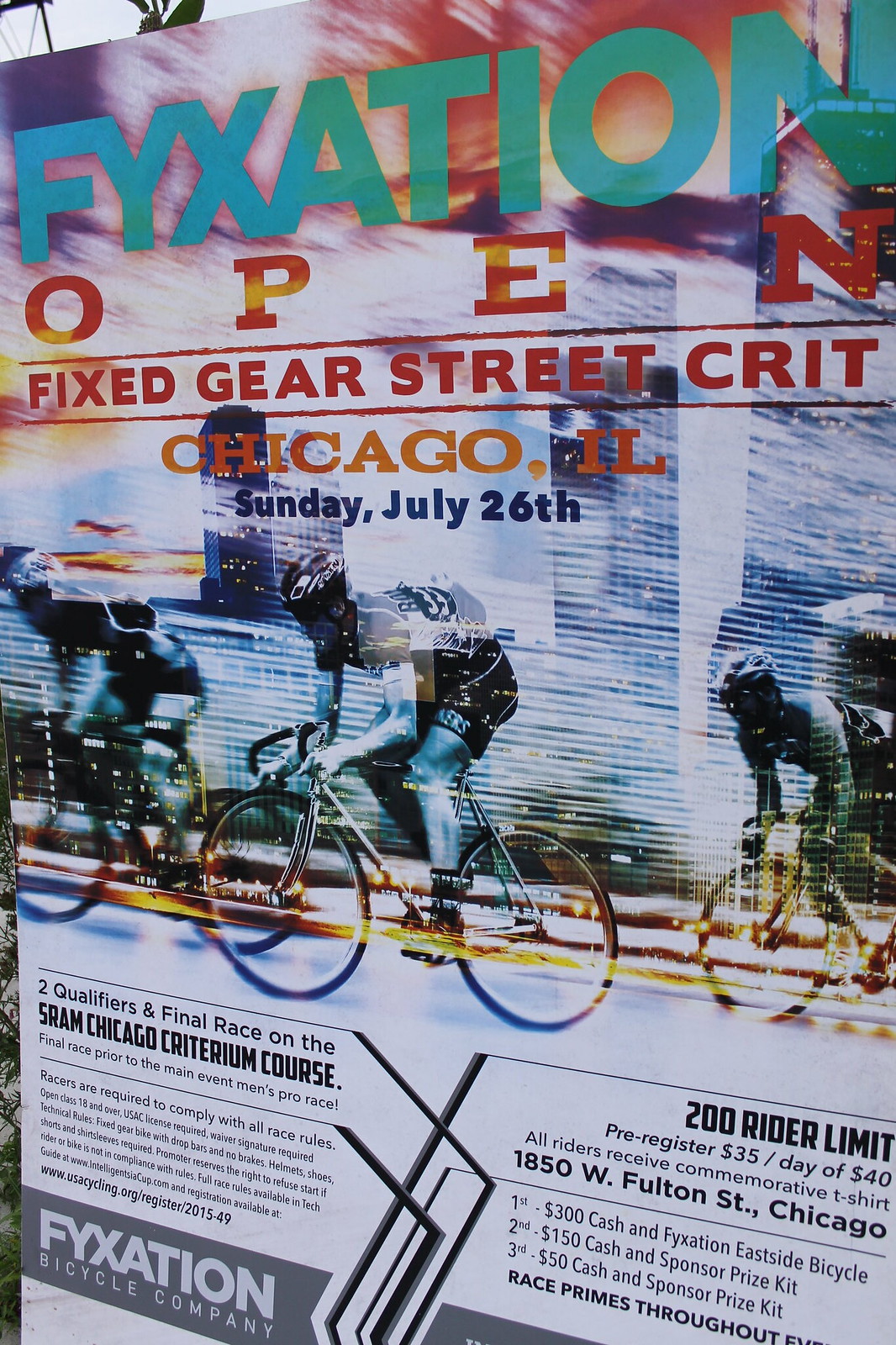This detailed poster promotes the Fixation Open, a fixed gear street criterium taking place in Chicago, Illinois. The header of the poster features the stylized text "Fixation," spelled F-Y-X-A-T-I-O-N in blue, below which "Open" is displayed in red. The tagline "Fixed Gear Street Crit" follows, albeit slightly cut off. The event is scheduled for Sunday, July 26th.

The central image depicts three fixed-gear cyclists racing against a blurred, stylized backdrop of the Chicago skyline, conveying a sense of speed and motion. Below the image, additional event information is presented in black text on a white background, divided into two columns. Details include:

- The race is held on the SRAM Chicago Criterium Course.
- There are two qualifiers and a final race.
- Men’s Pro Race has a 200 rider limit, with pre-registration costing $35 and day-of registration $40.
- All registered riders will receive a commemorative T-shirt.
- The race venue is 1850 West Fulton Street, Chicago.

Prize details are also outlined:
- First place: $300 in cash and a Fixation Eastside Bicycle.
- Second place: $150 in cash and a Sponsor Prize Kit.
- Third place: $50 in cash and a Sponsor Prize Kit.
- Additional race primes will be awarded throughout the event.